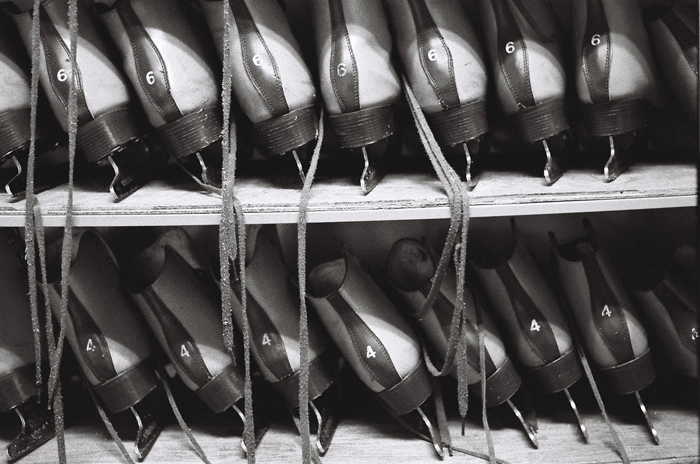This detailed black and white photograph captures the rental counter at an ice skating rink, showcasing two horizontal plywood shelves laden with ice skates. The top shelf holds an array of size six skates, identifiable by the number six painted on their backs. The skates are predominantly light-colored with a dark stripe, resembling the shape of a bowling pin, extending down the back. Their heels are also dark, adding to the striking contrast. Below, the second shelf displays size four skates, each marked with the number four on the back, and they seem to lean slightly to the left. Some of the laces dangle freely, adding to the scene's authenticity. The vintage style of the skates, reminiscent of Oxford shoes, is notable, with their flat metal blades and a combination of white bodies and black heels. The setting, likely a reception area for renting these skates, exudes a nostalgic charm through the simple, sturdy shelving and the orderly presentation of the skates.